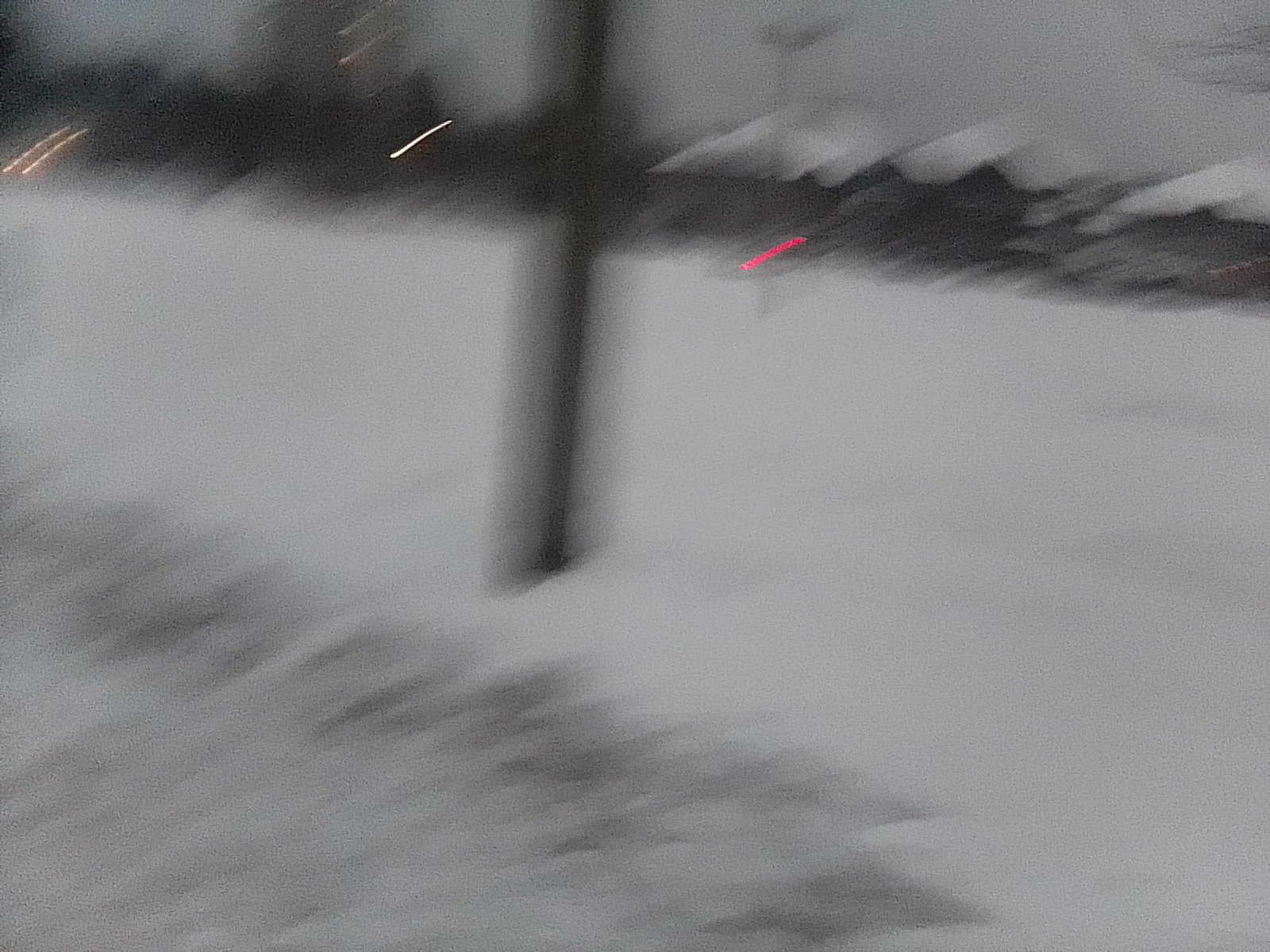The image, likely taken outdoors in motion, appears slightly blurry. Dominating the foreground is a black pole at the center, with another tall black pole visible to its right. A striking red line runs beside the central pole. To the left, there are distinct white and orange slashes. The scene is characterized by a large snowy field that covers most of the bottom and central parts of the image. The bottom left corner shows a darker shade of grey, where the snow seems to have been dirtied. The center is vividly white with jagged edges, leading up to roofs of houses in the background. These roofs are mostly white, likely covered in snow, forming triangular peaks. Above, the sky is entirely grey, dotted with thin, black wispy hair-like lines in the top right. Scattered drops in white, red, and blue hues suggest ongoing snowfall or rain. The overall impression is one of a snowy, overcast day with houses faintly visible behind what resembles a light dusting of snow and poles disrupting the scene.